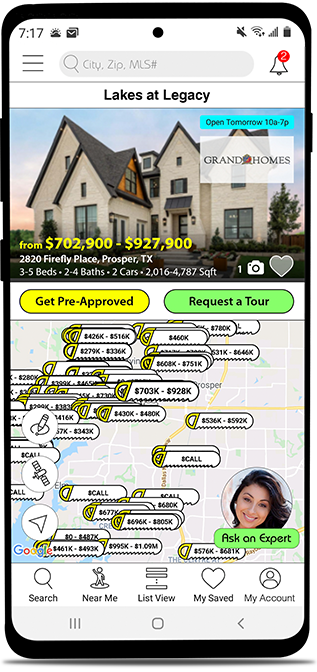Here is an improved and detailed caption for the described image:

---

The image shows a screenshot from an Android smartphone, likely highlighting a home listing. The screen's background is predominantly white at both the top and bottom. The top bar indicates the time as 7:17, with several notifications visible, including new email messages. To the right, icons display the phone's mute status, strong Wi-Fi signal, good reception, and a mostly full battery. On the far left, there is a hamburger menu icon, represented by three horizontal lines. Central to the top portion is a grayed-out search bar with a magnifying glass icon, allowing for searches by city, zip code, or MLS number.

Directly below this search bar is a thin gray line, beneath which, in bold black font with initial capitalization, are the words "Lakes at Legacy." The focal point of the image below this text is a vibrant photograph of an elegant home. A promotional banner states "Open Tomorrow 10am to 7pm," attributed to the real estate brand Grand Homes. The price range is highlighted in yellow as "From $702,900 to $927,900." Additionally, the address is clearly listed in white at the bottom of the image as "2820 Firefly Place, Prosper, Texas."

---

This detailed caption captures all essential elements and organizes them coherently for easy understanding.